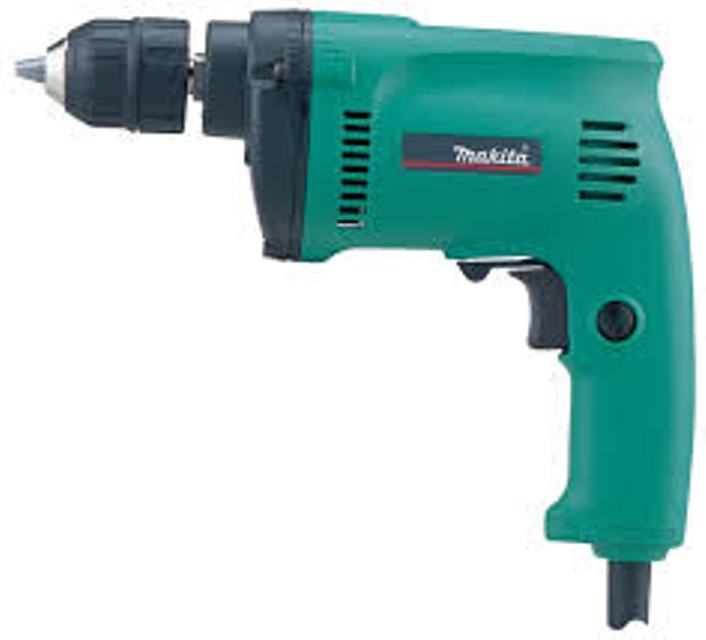The image appears to be an advertisement featuring a close-up, slightly blurry photograph of an electric power drill, showcasing a prominent side profile. The drill is primarily a sea green color, particularly on the handle and the initial section where the motor is housed. At the motor's end, there is a visible screw, suggesting the motor can be disassembled. The drill's front tip, including the replaceable drill bit, is black. The drill has a robust handle with a black trigger switch for activation. At the bottom, the beginning of a black power cord is visible. The brand name, "MAKITA," is printed in white on the drill, though parts of the label are somewhat difficult to read due to the image's quality. Additionally, the body of the drill seems to have vent-like openings likely for motor cooling and preventing overheating.